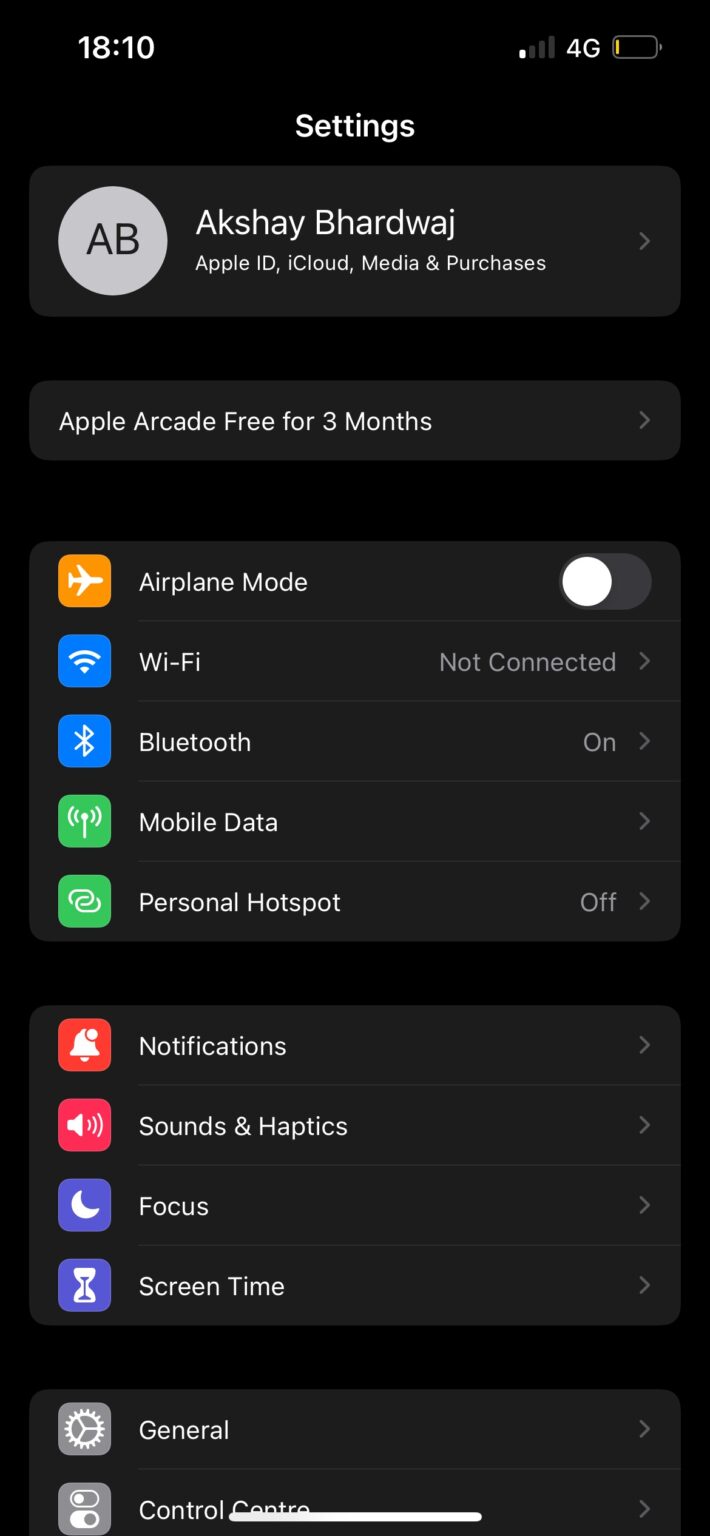This image is a screenshot of an iOS settings page, presented on a black background for enhanced contrast and readability. At the top center of the screen, "Settings" is displayed in white text. Just below, against a dark gray background, is a user profile section. This section shows an icon with the user’s initials or photo (if available) on the left, followed by the name "Akshay Bhardwaj" in white text. Directly beneath the name, a description reads "Apple ID, iCloud, Media & Purchases," accompanied by a clickable right arrow.

Further down, against the black background, a small dark gray section advertises "Apple Arcade free for three months" with a clickable right arrow to the right.

Next, a horizontally oriented, darker gray section houses five different settings options, each with its standard icon and label, all in white text:
- **Airplane Mode**: Set to off, indicated by a white slider button.
- **Wi-Fi**: Status shows as "Not Connected."
- **Bluetooth**: Status is on.
- **Mobile Data**
- **Personal Hotspot**: Set to off.

Following a brief black margin, another dark gray horizontally oriented section displays four settings options:
- **Notifications**
- **Sounds & Haptics**
- **Focus**
- **Screen Time**

Finally, glimpsed at the bottom of the truncated page, two more settings categories appear:
- **General**
- **Control Center**

Overall, this detailed screen captures essential user settings and options in neatly organized, color-contrasted sections for easy navigation.